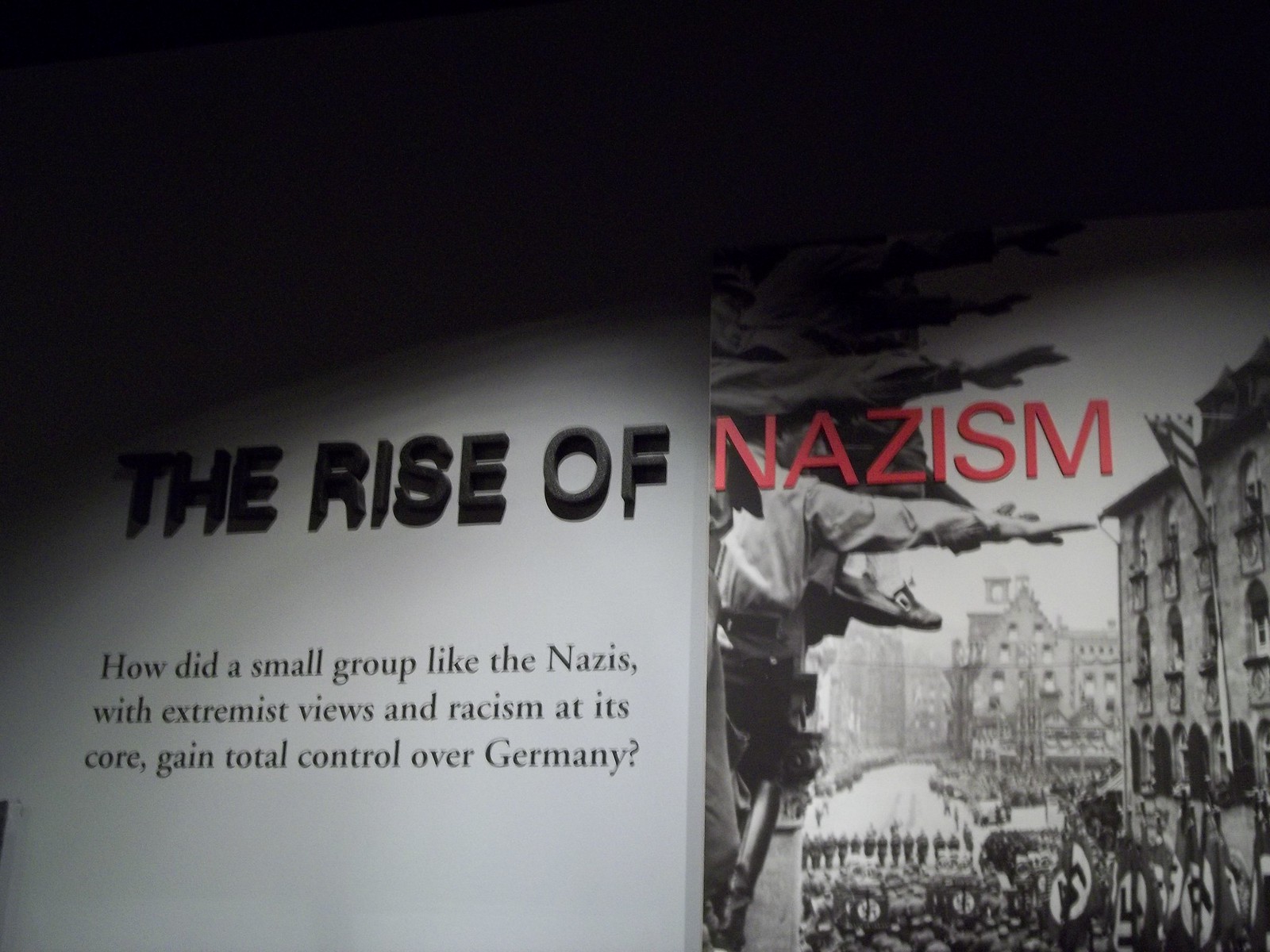The image depicts a detailed, black-and-white museum exhibit poster titled "The Rise of Nazism." The top of the poster is dark, featuring the phrase "The Rise of" in black metal letters, with "Nazism" prominently displayed in red over a group of people reaching their hands out from either a building or a railroad car, symbolizing the rise of Nazi ideology. The right side of the poster showcases an older granite building with windows, at the street level of which a Nazi parade, replete with prominent Nazi symbols, is taking place. In the background, another building with an arched roof is visible. The left side of the poster contains a thought-provoking question in black print on a gray background: "How did a small group like the Nazis, with extremist views and racism at its core, gain control over Germany?" This museum exhibit sign is likely part of a larger display, possibly in a World War II museum, that guides visitors through the historical events surrounding the rise of the Nazi regime.